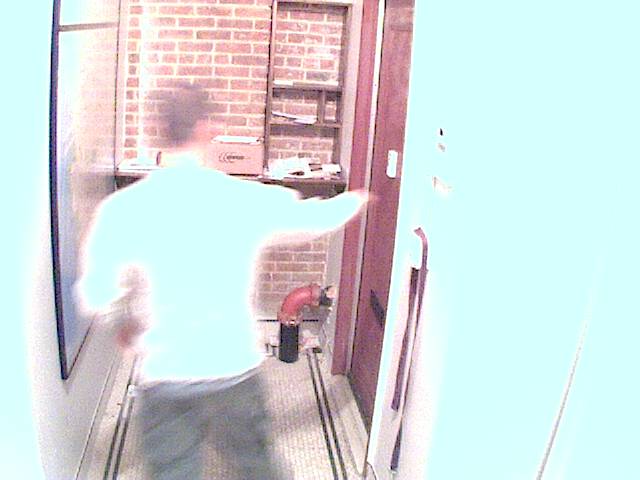In this photograph, we see a man silhouetted against a brightly lit hallway, giving the image an overexposed, almost surreal quality with washed-out colors that take on a sky-blue hue. He stands facing a brownish-red door to his right, reaching out with his right hand as if intending to enter. The man, dressed in a slightly blurred sky-blue or light-colored top and gray pants, has short dark hair. The hallway features a tan carpet accented with black stripes and exposed bottom pipes. 

Behind him is a brick wall in shades of brown, adorned with wooden shelving that holds a variety of items including a package with a newegg.com logo and several envelopes, suggesting it might be a mail delivery area, potentially within an apartment complex. The overwhelming brightness of the photograph creates an impression of a digital or virtual game environment, further obscuring finer details but highlighting the scene's unique atmosphere.